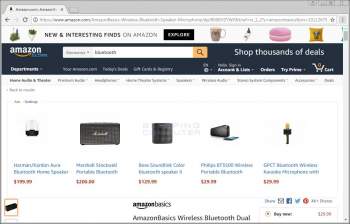The web page displayed is compact and the text is minuscule, making it challenging to read. The header at the top of the page reads "New and Interesting Finds on Amazon." The layout includes various small images, among which the only clearly recognizable one is a mug. The page also promotes "Thousands of Deals." The other images are somewhat ambiguous: one appears to be a transparent glass object with a black base, another is a black rectangle with small spots on it, there's a barrel-shaped item with straight sides, and what looks like a television screen. There is also another unclear object that is difficult to identify.